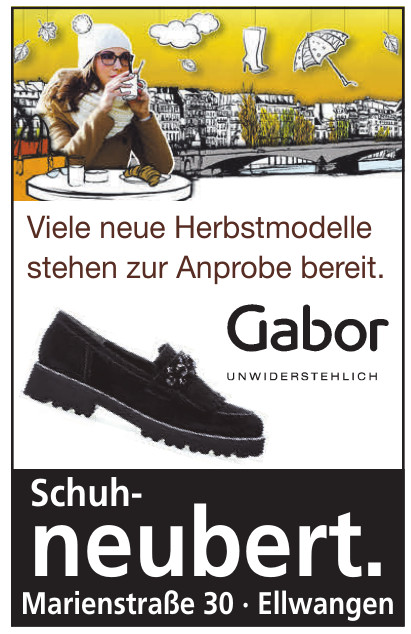The image is an advertisement, likely a poster or magazine page, for a store or cafe. Dominating the top section of the image is a photorealistic woman dressed in winter clothing: a white hat, white scarf, tan jacket, and black-framed glasses. She is seated at a small, cartoonishly illustrated table, sipping from a white cup while a croissant and a glass of milk or water sit in front of her. Behind the woman, an intricately drawn cityscape unfolds, featuring buildings, a gray bridge, and trees shaded in yellow, brown, and green, all against a golden-yellow sky. Dangling from the sky are illustrations of an umbrella, a leaf, boots, and clouds, hanging from wires.

In the middle of the image, a black shoe is showcased diagonally, with "Gabor" prominently printed in black text to its right, surrounded by additional foreign language text. The shoe itself is dark blue, extending to a dark gray heel of over an inch. The background transitions from yellow at the top, to white in the middle, and to black at the bottom, where the white text, likely German, lines the lower part of the poster. The entire image is framed by a thin black line, adding to the structured aesthetic of the advertisement.